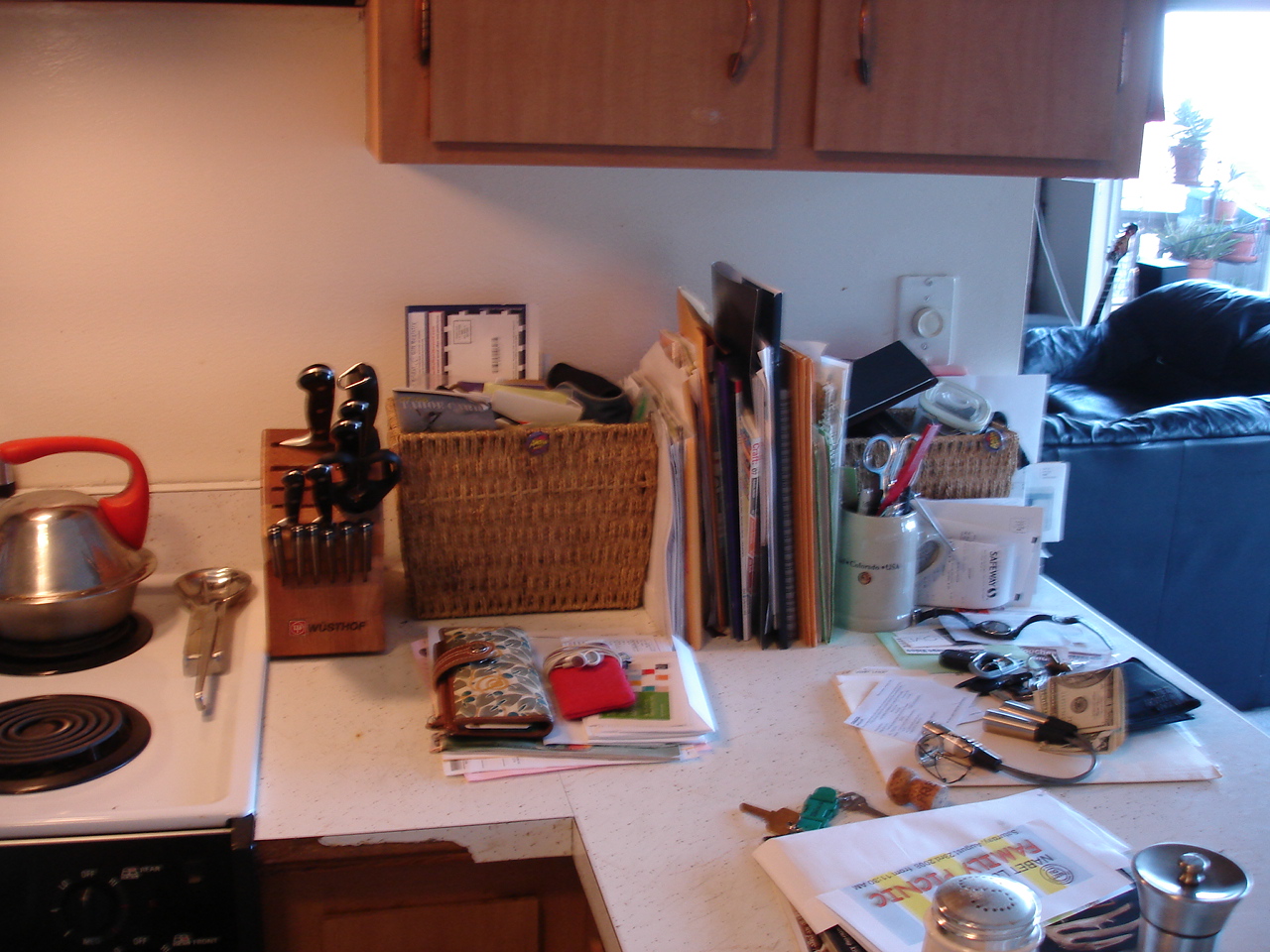The image displays a cluttered countertop in an open kitchen that seamlessly leads into a living room area. The living space features a piece of black leather furniture, likely a personal chair, with a smooth side and a wrinkled top. Positioned by a door that appears to provide access to a patio, there is a guitar standing upright. This patio area is adorned with various potted plants, adding a touch of greenery.

In the kitchen, a single brown cabinet with two handles is noticeable against a white wall backdrop. Below, a stove with a tea kettle featuring an orange handle subtly stands out. The countertop itself is a hub of activity; it holds a wallet, a phone, some money, and possibly headphones. Central to the countertop is a collection of paper envelopes and other assorted items, organized amidst two baskets filled with miscellaneous objects.